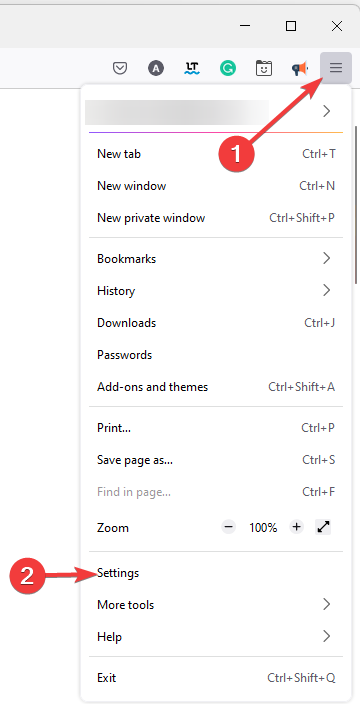Here is a screenshot of a web browser with a dropdown menu expanded to reveal additional options and settings. The browser interface resembles popular browsers such as Chrome, Explorer, or Firefox. In the upper right-hand corner, within a gray border, are the minimize, maximize, and close buttons. 

Adjacent to these buttons are extension icons labeled "A," "LT," "G," a smiley face, and a megaphone, followed by a three-bar menu icon with a red arrow and the number one. Clicking this icon opens a dropdown menu with the following options: New Tab, New Window, New Private Window, Bookmarks, History, Downloads, Passwords, Add-ons and Themes, Print, Save Page As, Find in Page, Zoom (with options for -100% and +), and an Expand button.

Additionally, there is a red circle with the number two and an arrow pointing to a "Settings" button. Further options in the dropdown include More Tools, Help, and Exit. Several of these options have keyboard shortcuts for quick access, such as Control + T for New Tab, Control + N for New Window, Control + Shift + P for New Private Window, Control + P for Print, Control + F for Find in Page, and Control + Shift + Q for Exit.